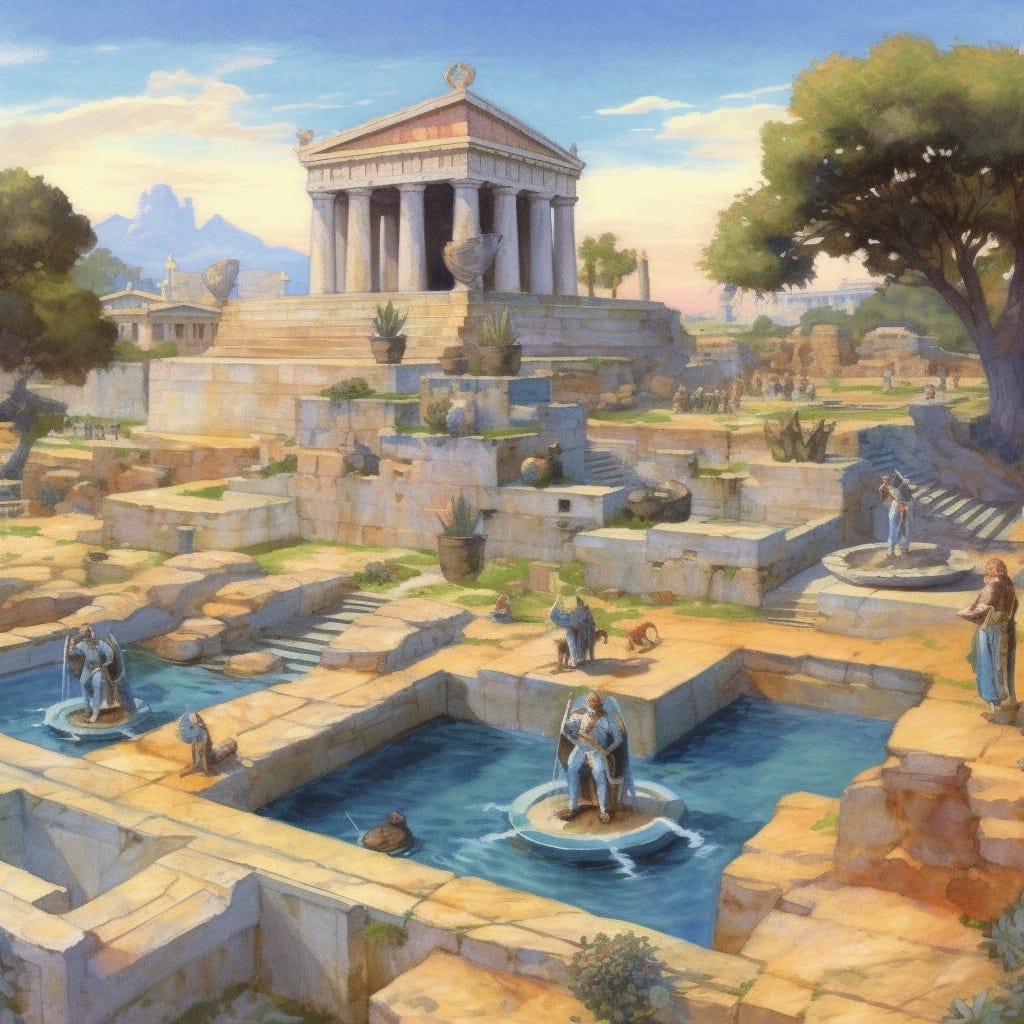This detailed image appears to be a hand-drawn or computer-animated artwork with a smooth digital style. Central to the scene is a grand, ancient Roman-style temple or coliseum, prominently elevated and featuring seven towering columns with a triangular pediment at the top. The temple is surrounded by numerous sections of stone structures, primarily in cream, orange, rust, yellow, tan, and gold tones, forming a labyrinth-like design. Stone steps descend from the temple into various baths and pools of blue water, each adorned with statues pouring water into the pools.

In the foreground and along the edges of these pools, stone walls create separate sections, each decorated with urns and potted plants, suggesting a rich, historical atmosphere. Guardian figures, possibly statues of soldiers, are positioned on these walls. The background features a picturesque outdoor setting with a bright blue sky dotted with white clouds. Trees are intermittently placed, particularly evident in the upper right corner, enhancing the natural backdrop of this ancient cityscape. The entire composition exudes the grandeur and architectural brilliance of ancient Rome.